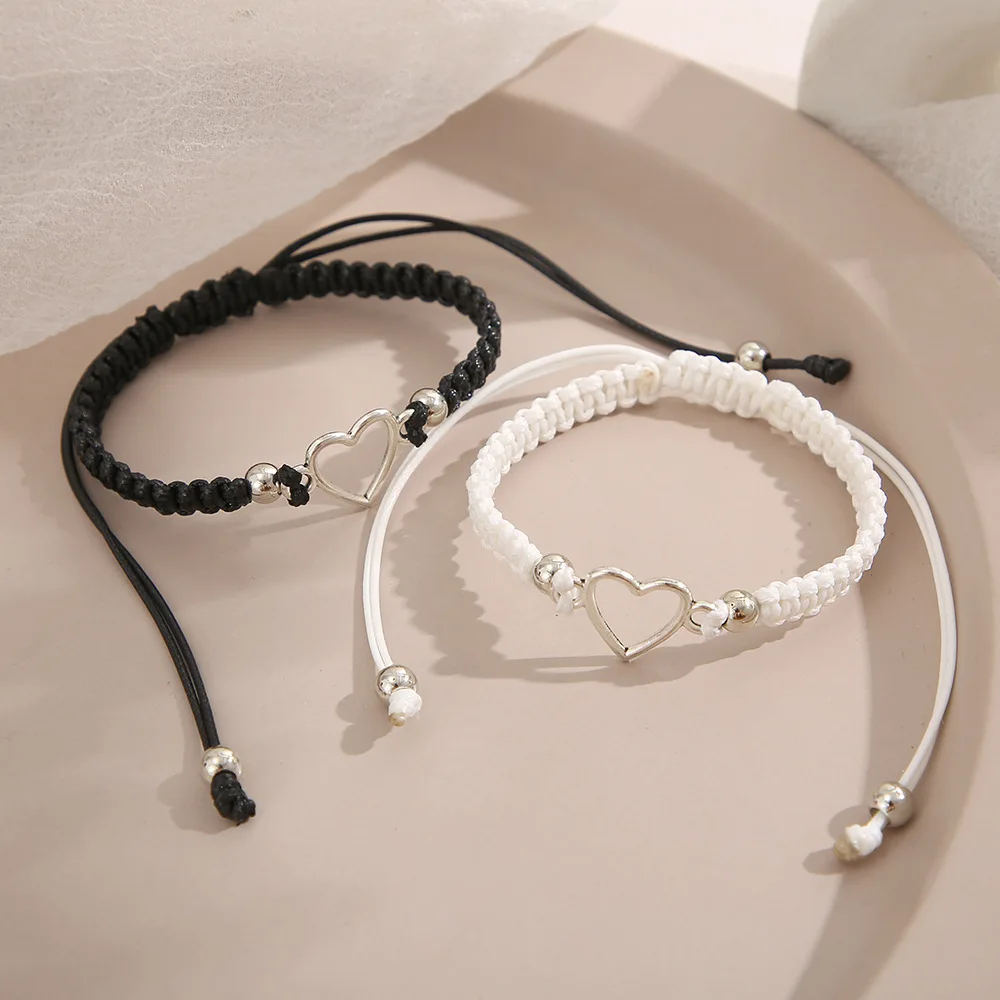The image displays two intricately designed braided bracelets, placed on a light tan-colored leather surface, possibly a desk chair. Both bracelets share a similar design, featuring a central silver heart-shaped medallion. The bracelet on the left is crafted from black braided nylon, while the one on the right is made from white braided nylon. Each bracelet includes silver beads located near the connecting heart pendant and at the ends of the drawstrings, which allow for adjustable sizing. Additionally, the drawstrings, black for the black bracelet and white for the white bracelet, extend from the central heart medallion. The background also includes hints of a white backing in the upper left corner and armrests on the upper right, contributing to the overall setting.